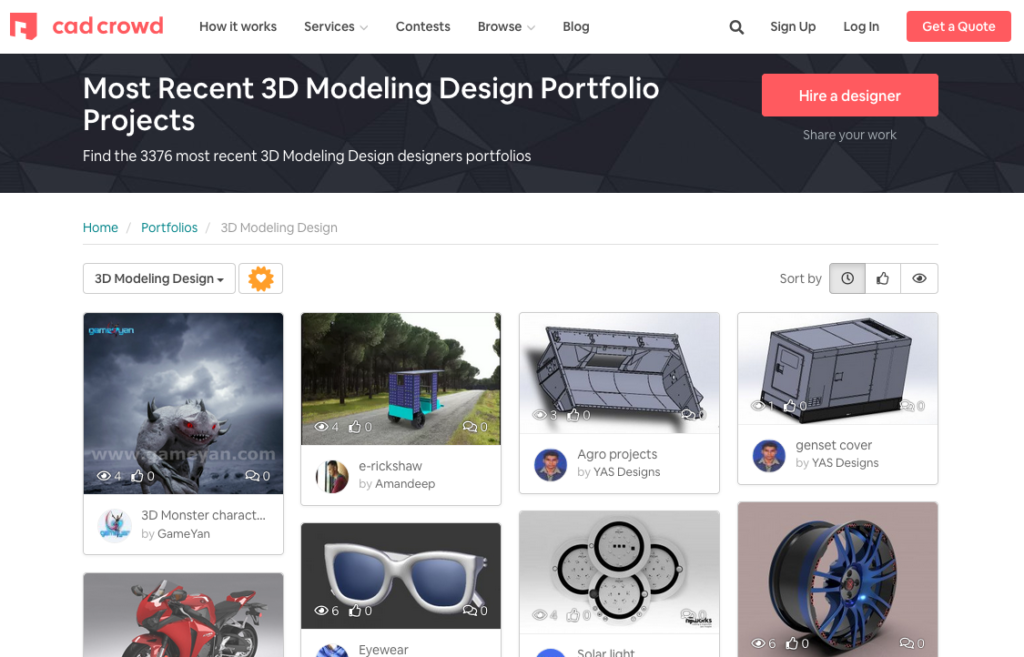The screenshot captures the homepage of the CadCrowd website, showcasing its layout and design elements. In the top left corner, the CadCrowd logo is prominently displayed. Adjacent to the logo on the right, there are five main navigation categories listed: "How It Works," "Services," "Contests," "Browse," and "Blog." Towards the far right of the header, there is a search icon represented by a magnifying glass, alongside options to "Sign Up," "Log In," and a bold, red "Get a Quote" button with white text.

Below the header, a large black banner spans the width of the page, featuring a prominent message in big white letters: "Most Recent 3D Modeling Design Portfolio Projects." Directly beneath this, smaller white text reads: "Find the 3,376 most recent 3D modeling designers portfolios." To the right of this banner, there's a substantial red rectangle button labeled "Hire a Designer" in white font. Beneath this button, a subtle prompt in small white text encourages users to "Share your work."

The main body of the website, which features a white background, starts immediately below the banner. At the top of this section, navigation links for "Home," "Portfolios," and "3D Modeling Design" are visible. A dropdown box is set to "3D Modeling Design," indicating the current content focus. The page displays thumbnails of 3D designed images, arranged in two rows of four thumbnails each. It is worth noting that the bottom portion of the second row of thumbnails is cut off due to the screenshot being cropped.